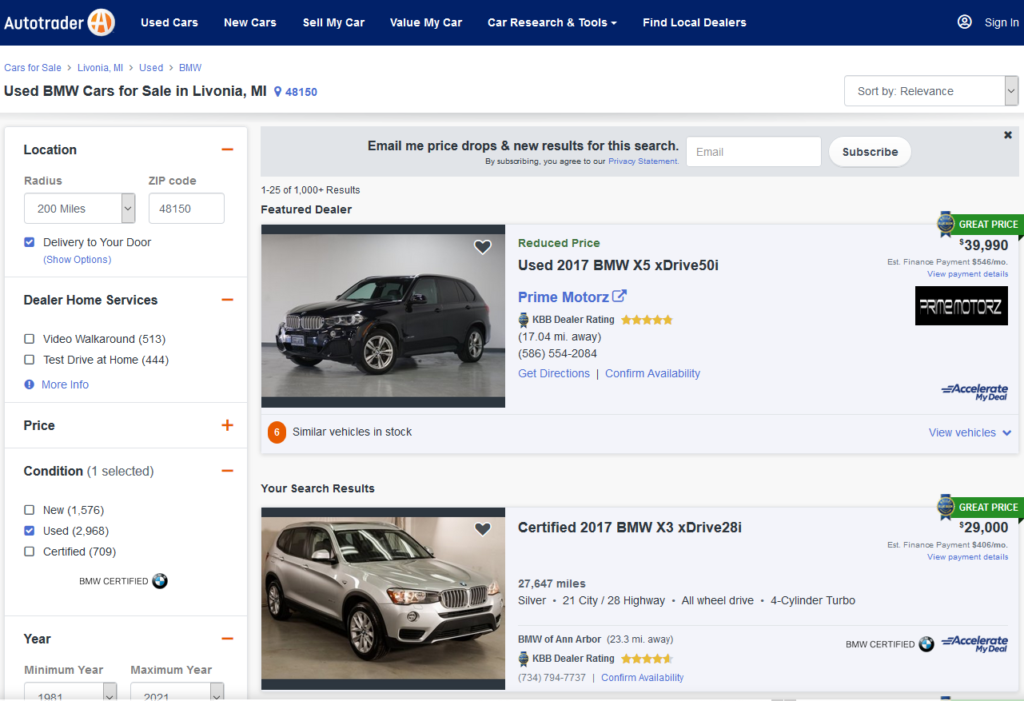The image displays a webpage from AutoTrader. At the top, there's a national banner featuring white text. The primary text within the banner reads "AutoTrader" in larger white print, complemented by an adjacent orange circle with a white 'A' inside. Directly beneath this, the navigation menu items are listed in white text: "Used Cars," "New Cars," "Sell My Car," "Value My Car," "Car Research and Tools," and "Find Local Dealers," followed by a "Sign In" option.

The main content area of the webpage has a white background and a blue text header that reads "Cars for Sale, Livonia, Michigan, Used BMW." This is followed by a bold, black title: "Used BMW Cars for Sale in Livonia, Michigan. Zip Code 48150." On the right-hand side of this section, there's a sorting option labeled "Sort by: Relevance," featuring a gray bar with a downward arrow.

A sidebar on the left side of the page, displayed in white, lists various filter options: "Location," "Other Home Services," "Price," "Condition," and "Year." At the top of this sidebar, a gray banner offers functions for email notifications: it reads "Email Price Drops and New Results for This Search" and includes a field for users to enter their email address, accompanied by a "Subscribe" button.

Further down the page, two images are shown side by side, each depicting a different car. Each image is paired with detailed descriptions and relevant information about the respective vehicles.